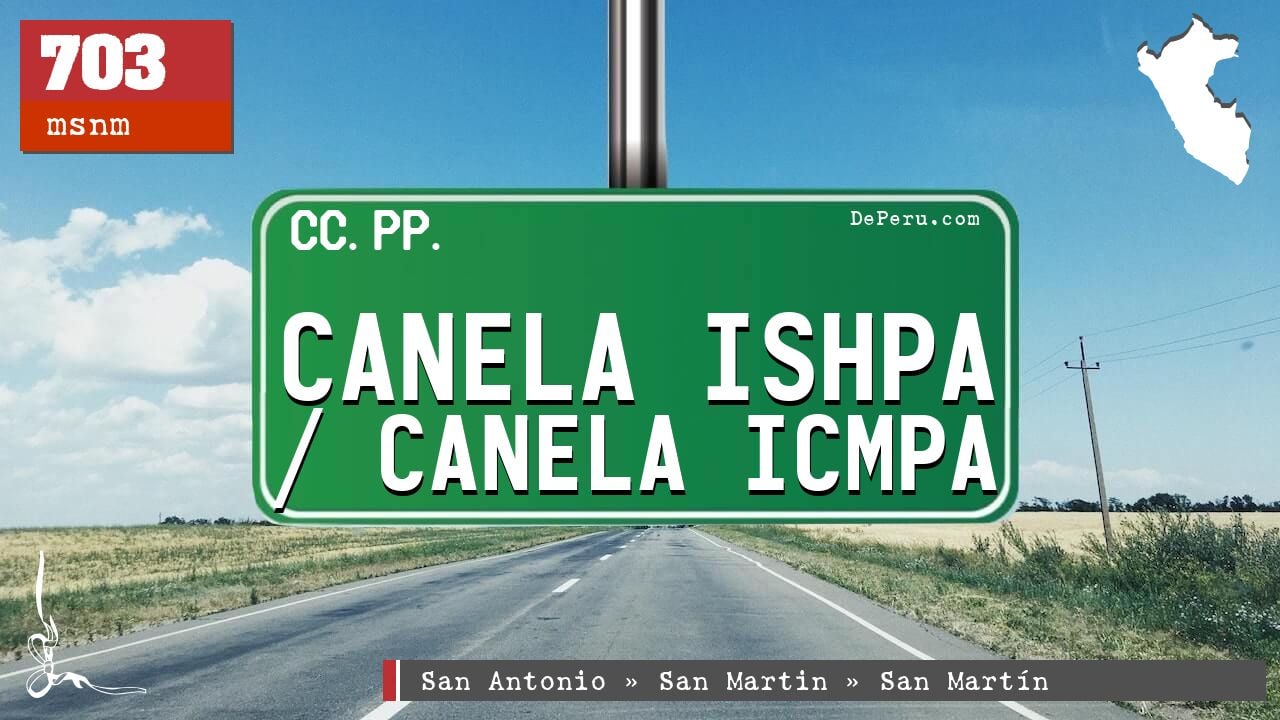The image captures a snapshot from the dashboard of a car driving on an empty, sunny, two-lane country road. A green road sign prominently displays "Canela Ixpa" and features a web address "ferru.com" alongside. There's a red box to the left of the sign that reads "703 MSNM," and overhead wires run along the roadside. The sky is blue with scattered clouds, and fields stretch out on either side of the road. In the top corner of the image, the words "D-E Peru" are visible, suggesting a Peruvian location. An outline on the sign resembles a country, hinting at either European or South American geography. The serene setting and clear weather emphasize the rural nature of the scene.